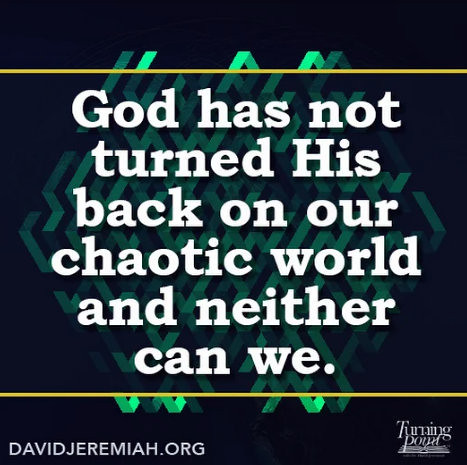The image is a square poster with a predominantly black background featuring a central, bold, inspirational message in white text: "God has not turned his back on our chaotic world and neither can we." This text is written in a serif font, likely Georgia. Separating the text are horizontal gold stripes, creating a bordered effect above and below the text. Behind the words, there's a shiny green design with a Middle Eastern or Far Eastern pattern that adds a subtle but vibrant element to the background. In the lower left-hand corner, the URL "davidjeremiah.org" is displayed in all capital letters, rendered in a sans-serif font. In the lower right-hand corner is the logo of the organization "Turning Point," characterized by a capitalized and italicized "T" and the rest of the word "point" in lowercase italics, accompanied by an image resembling a turning book spine.